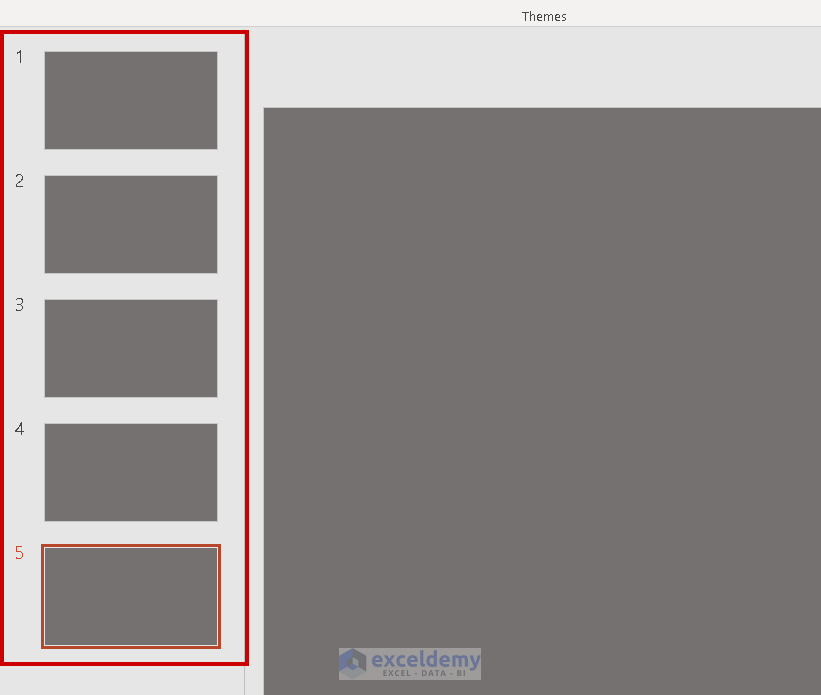Here is a cleaned-up and detailed caption for the image described:

---

The image displays a predominantly blank screen set against a light gray background. At the very top of the screen, there is a thin bar that contains a few themes. Positioned in the middle of the screen is a divided layout with two sections. 

On the left side, there is a section outlined in red. This section comprises five vertically arranged gray boxes, numbered 1 through 5. Notably, the fifth box is also specifically outlined in red.

On the right side, a much larger gray box dominates the space. In the bottom left corner of this larger box, a small logo is visible. The logo includes the name "Exildemi" and features a hexagonal emblem composed of blue, black, and light blue segments. Below the "Exildemi" text, there is smaller text that reads "Excel-Data-BI" or something similar.

---